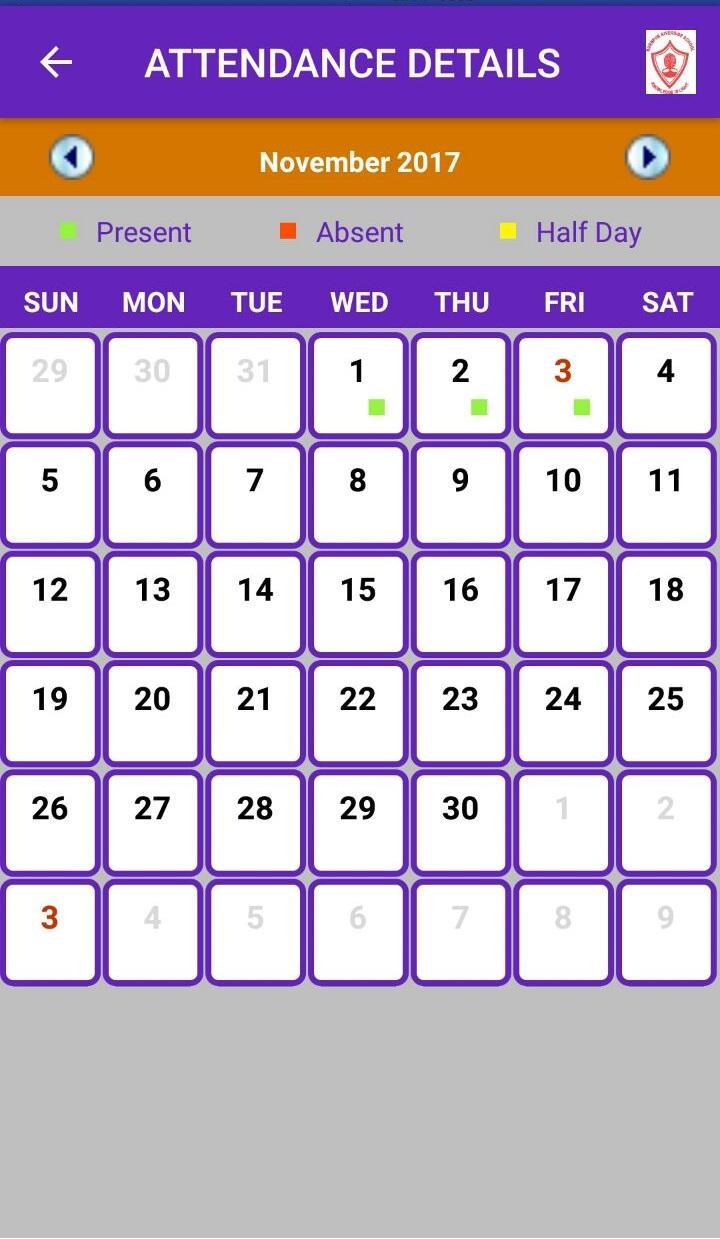A screenshot of an attendance-tracking app interface is displayed. At the top of the screen, the heading "Attendance Details" is prominently featured in purple, with the date "November 17th" just below it. Arrow icons are present to allow users to cycle through different calendar dates. The calendar view spans from the 29th of the previous month to the 9th of the current month, November 17th. Each date is encased in a purple, rounded rectangle with a white background inside the borders. 

Attendance statuses are color-coded: green indicates "Present," red signifies "Absent," and yellow denotes a "Half Day." Only three specific dates—November 1st, 2nd, and 3rd—are marked with these attendance statuses, providing a clear visual record of attendance.